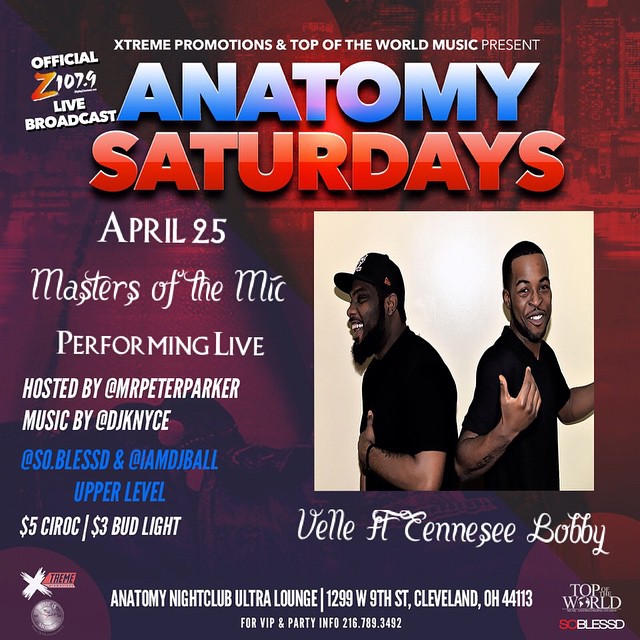The vibrant poster titled "Anatomy Saturdays" is tinted in a striking combination of red and purple hues, with a background image that appears to depict city buildings subtly visible in the top right corner. Prominently positioned in the center-right of the poster is a square photograph featuring two black men, joyfully smiling and laughing, with the man on the left looking to the side and the man on the right facing forward. Above the photo, the text reads "Anatomy Saturdays" in blue and red fonts, respectively, and "Extreme Promotions and Top of the World Music Present" in a smaller font above. 

This event, scheduled for April 25th, highlights "Masters of the Mic Performing Live" hosted by Mr. Peter Parker, with music provided by DJ KNYCE, SO.BLESSD, and IAMDJBALL. The night promises $5 Ciroc and $3 Bud Light at the upper level of the Anatomy Nightclub Ultra Lounge, located at 1299 West 9th Street, Cleveland, Ohio, 44113. Additional details include an official Z107.9 live broadcast and VIP/party information available by calling 216-789-3492. The names V-E-L-L-E, F-L, C-E-N-N-E-S-E-E, and Bobby are mentioned beneath the photograph, indicating possible performers. The poster captures a wealth of information about this lively event, promising a memorable night of live music and entertainment.